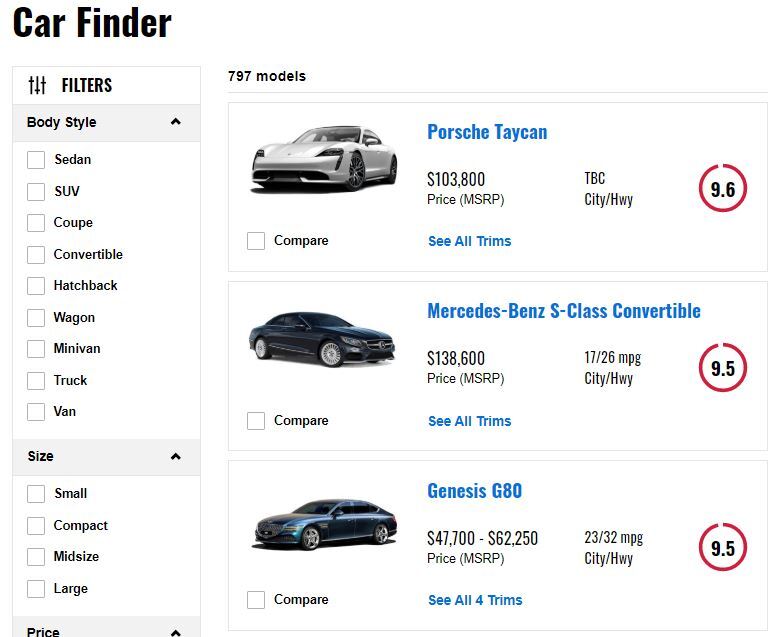The image is a screenshot likely taken from a desktop website specializing in automobiles. At the top of the page, the words "Car Finder" are prominently displayed in black ink. Below this heading, a series of filter tables are presented to help refine the car search. 

The first table is labeled "Filters" and allows users to choose a body style from options such as sedan, SUV, coupe, convertible, hatchback, wagon, minivan, truck, or van—all written in black ink. As depicted in the screenshot, no body styles have been selected. 

Following this, there is a filter for size, offering choices like small, compact, mid-size, and large. There's also a filter for price, although this part of the screen is cut off and not fully visible.

The page displays a total of 797 car models. The first car shown is a grey Porsche Taycan, priced at $103,000. Next to it, a red circle contains the number "96" in black ink, though the significance of this number is unclear. The second car is a black Mercedes-Benz C-Class Convertible, listed at $138,600. The final car is a Genesis G80, which appears to be dark green, though the exact color is uncertain. 

Each car's name is written in blue ink, as is the link "See All Trims," which offers additional options for each model.